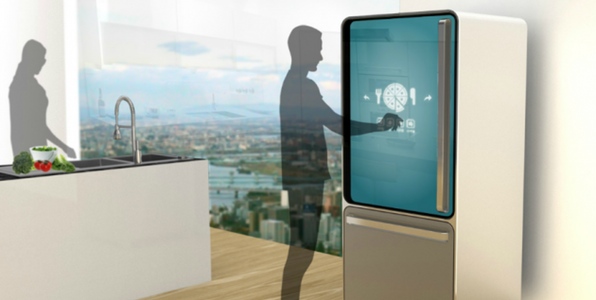In this horizontally aligned rectangular image, we have a detailed, AI-generated depiction of a modern kitchen set in a high-rise apartment with a large window overlooking a vast cityscape. The scene is bathed in light coming from the window, highlighting the hardwood floors that are a light brown, almost beige color. 

In the kitchen, there is a central island with a black countertop. On the left side of this island, a metallic curved faucet extends over a sink, which is divided into two sections. Above the sink are some brightly colored vegetables, including red tomatoes and green vegetables, sitting in a white bowl.

On the far right side of the image, there is a white refrigerator with a blue touchscreen on the door. Below the screen, there's a horizontal bar indicating the freezer section with a gray background. The fridge also features a vertical metal handle on the door and a smaller handle at the bottom for the freezer compartment. The window captures a scenic view of the city, with outlines of distant buildings and a glimmering body of water under a somewhat blurred sky.

Silhouetted in dark, translucent black are two people, their semi-transparent figures adding a touch of activity to the kitchen. The man, positioned near the fridge, appears to be pressing the blue touchscreen, possibly ordering food, given the white pizza emblem displayed on the screen. The woman, located on the left side of the image, seems to be cutting vegetables on the countertop. Their shadows merge harmoniously with the serene, modern kitchen setting, providing a subtle yet dynamic human presence in the scene.